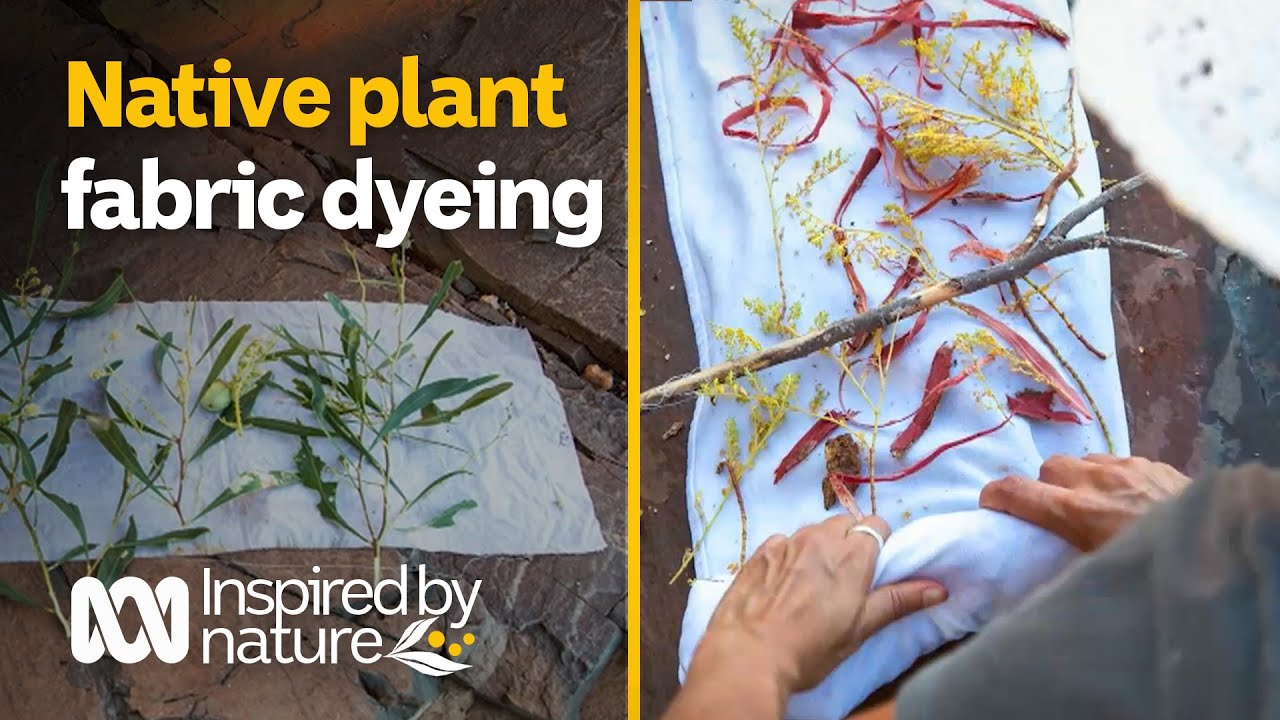The image, resembling a tutorial or instructional guide, is split into two sections by a bold yellow line. On the left side of the image, a photograph angled downward shows a white cloth laid across a rocky ground. Green leaves and stems are spread along the length of the cloth. At the top, in a large orange-yellow font, it reads "Native Plant," followed by "Fabric Dyeing" in white text, and at the bottom, the phrase "Inspired by Nature" is written, accompanied by two white leaves with three yellow circles resembling pollen or seeds.

The right side features another fabric, this time positioned vertically, with various yellow and red leaves, stems, and a brown stick placed on top. A person, identifiable by a gray shirt, a hat, and a ring on the left-hand pointer finger, is shown rolling up the cloth with the plant materials inside from the bottom. The composite visuals and text create a detailed advertisement for fabric dyeing inspired by natural elements.